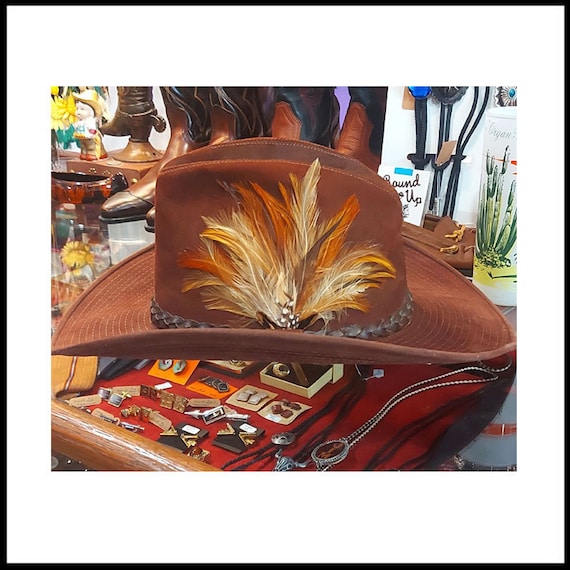This image features a framed square photograph, bordered in black with a white matte, capturing the vibrant essence of a western store display. At the center of the image is a large, rustic, copper-colored cowboy hat. The hat, made of brown suede-like material, is adorned with a slender band that resembles snake skin, and embellished with a multitude of feathers. Dark feathers encircle the base while larger feathers in shades of orange, tan, and white embellish the side. The hat rests on a glass countertop, beneath which an array of jewelry items such as earrings, necklaces, cufflinks, and bolo ties with silver and turquoise buckles are visible. Behind the hat, several pairs of cowboy boots are displayed, and a small figurine and flower ornaments add an eclectic touch to the background. To the upper left, a cowboy boot mounted on a metallic pedestal can be seen, and to the upper right, a sign reading "Roundup" is visible, enhancing the western theme. A glass adorned with a cactus motif also rests on the counter, adding to the detailed setting of this intriguing storefront.